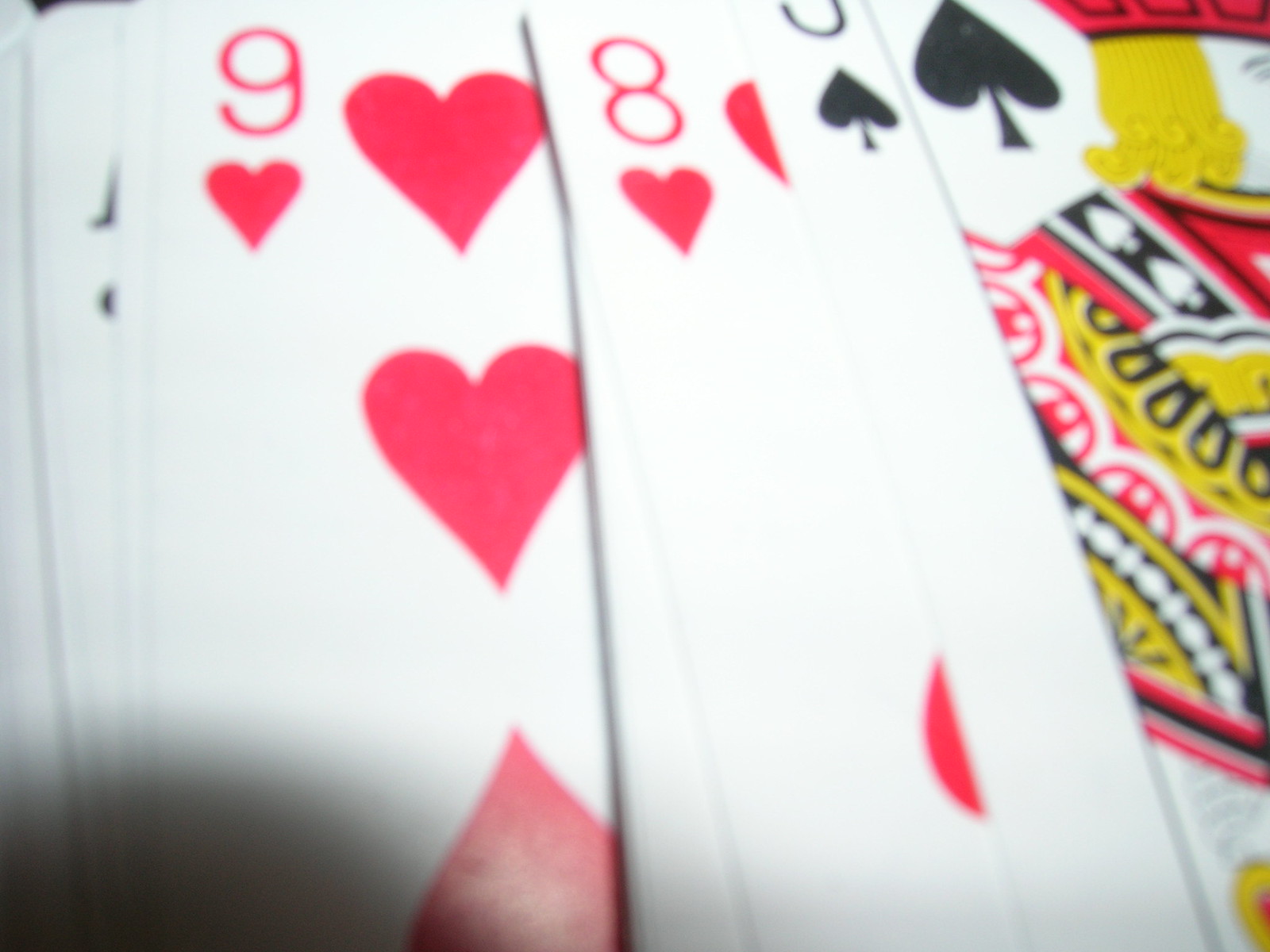This is an extreme close-up, color photograph of a partially visible array of playing cards, arranged in an overlapping manner that suggests either a shuffle or a spread for a magic trick. The image is in landscape format and is notably blurry and pixelated, contributing to its low resolution. The cards are cropped by the edges of the frame, eliminating any background and preventing a full view of any single card. Dominating the left side is a nine of hearts, with an eight of hearts partially overlapping it. Toward the right, the jack of spades slightly crops out with its vibrant red, white, black, and yellow robed character and red crown, though the face remains unseen due to the cropping. Additionally, there is a probable ace of spades barely visible and other indistinct cards suggesting further depth in the array. The arrangement of the cards appears slightly spaced apart, though still significantly overlapping.